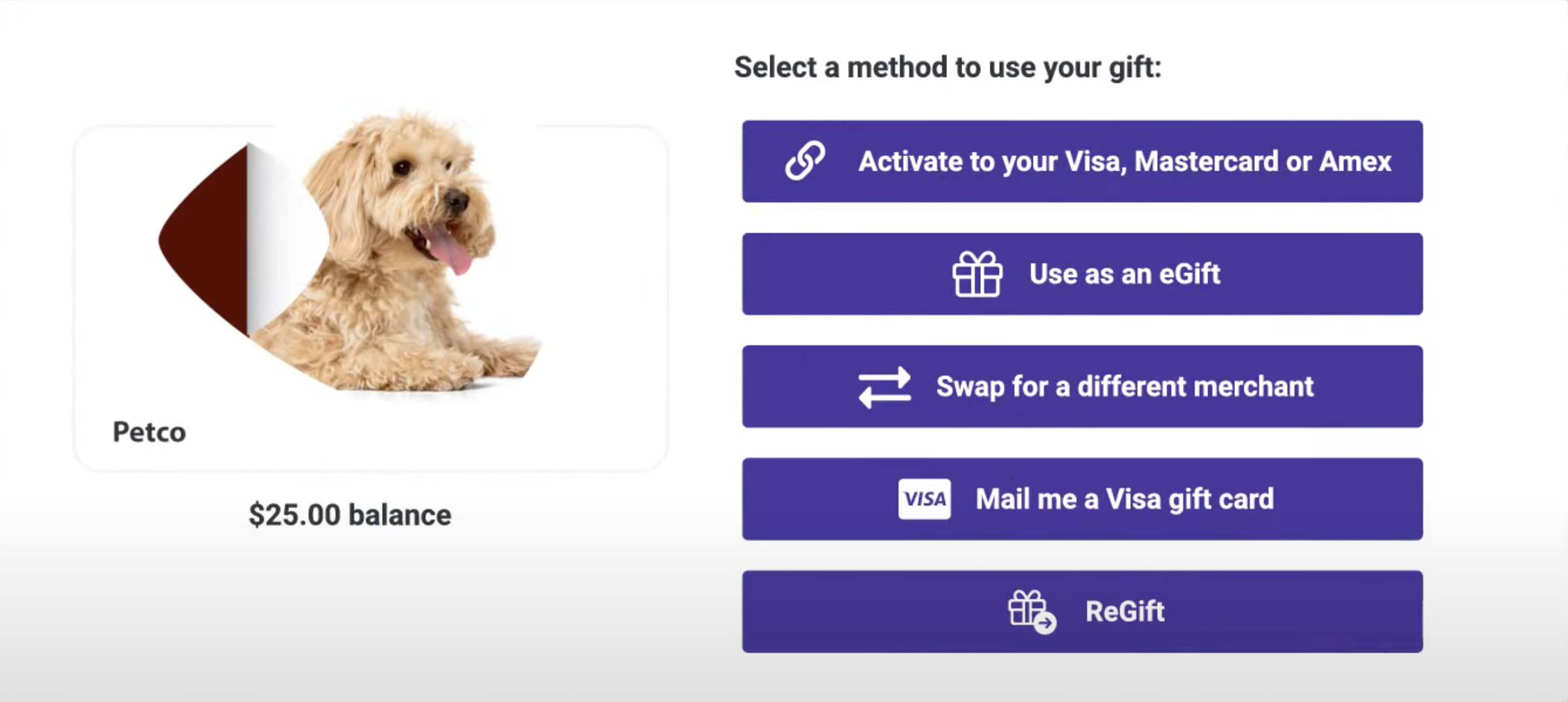The image displays a webpage with a white background, subtly transitioning to grey in the bottom right corner. On the right side of the page, there are five prominent, vertically aligned purple buttons with white text, each representing a method to use "Kibs." At the top of these buttons, a header reads: "Select a method to use your Kibs."

1. The first button reads, "Update your Visa, Mastercard, or Amex," accompanied by an icon of a chain.
2. The second button says, "Use as an e-gift," featuring an icon of a gift.
3. The third button indicates, "Swap for a different merchant," with an icon showing two arrows pointing in opposite directions.
4. The fourth button reads, "Mail me a Visa gift card," marked with a Visa icon.
5. The fifth and final button is labeled, "Re-gift," and is indicated with an icon of a gift and an arrow.

On the left side of the page, there's a picture of a dog with brown fur and its tongue sticking out. Below the dog picture, the brand name "Petco" is displayed, and further below, there's text indicating a price, "25 per land," written in black. The layout and structure suggest thoughtful organization and clarity, ensuring that users can easily navigate and understand their choices for utilizing their Kibs.